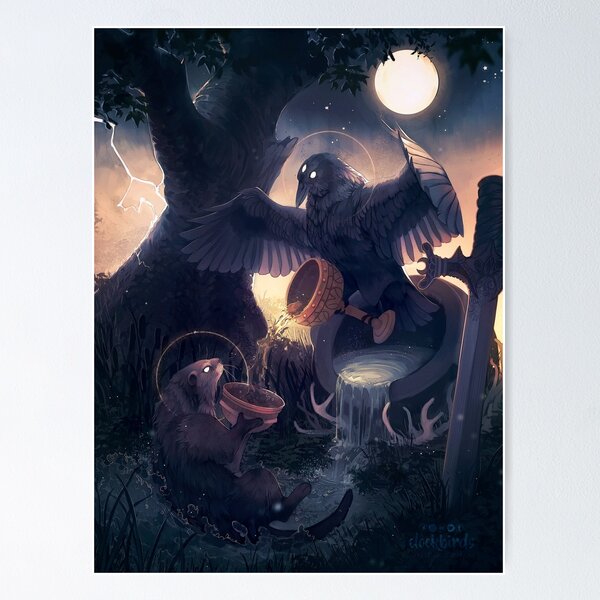In this detailed gothic-style illustration set at night, a dark, three-eyed raven with an additional eye on its forehead and eyes depicted in side profile stands amidst a surreal, partially water-logged landscape. The raven grips a golden chalice in its feet, gracefully pouring liquid into a golden chalice held by an attentive otter or beaver. Behind them, a mysterious cauldron gushes water that swirls around the base of a large, knotted, and ancient tree. The scene is illuminated by a glowing, solid yellow moon hanging prominently in the top right corner of the composition, casting eerie light over the tableau. Lightning bolts streak the orange-tinted sky in the background, adding to the dramatic and enigmatic atmosphere. A dagger or sword is firmly embedded in the ground, enhancing the mystical aura. The entire setting evokes a sense of dark, fantastical symbology and profound, perhaps arcane, meaning.